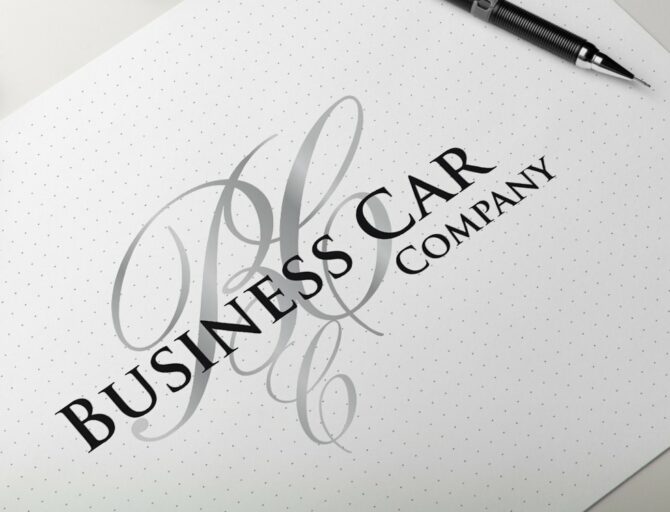The image showcases a diagonally placed business card against a predominantly white background with a solid medium gray color peeking through the upper left, upper right, and lower right corners. The card itself features a textured pattern of tiny gray dots reminiscent of lattice work. Centered on this white card, a stylish logo consisting of the letters "BC" is depicted in a decorative, silvery gray script. Superimposed over this logo, in bold black capital letters, are the words "BUSINESS CAR COMPANY." In the upper right corner of the image, the tip of a black mechanical pencil with a silver tip and visible lead appears, suggesting an elegant touch but not meant for writing on the card. The entire setup gives the impression of a meticulously designed digital image rather than a traditional photograph.